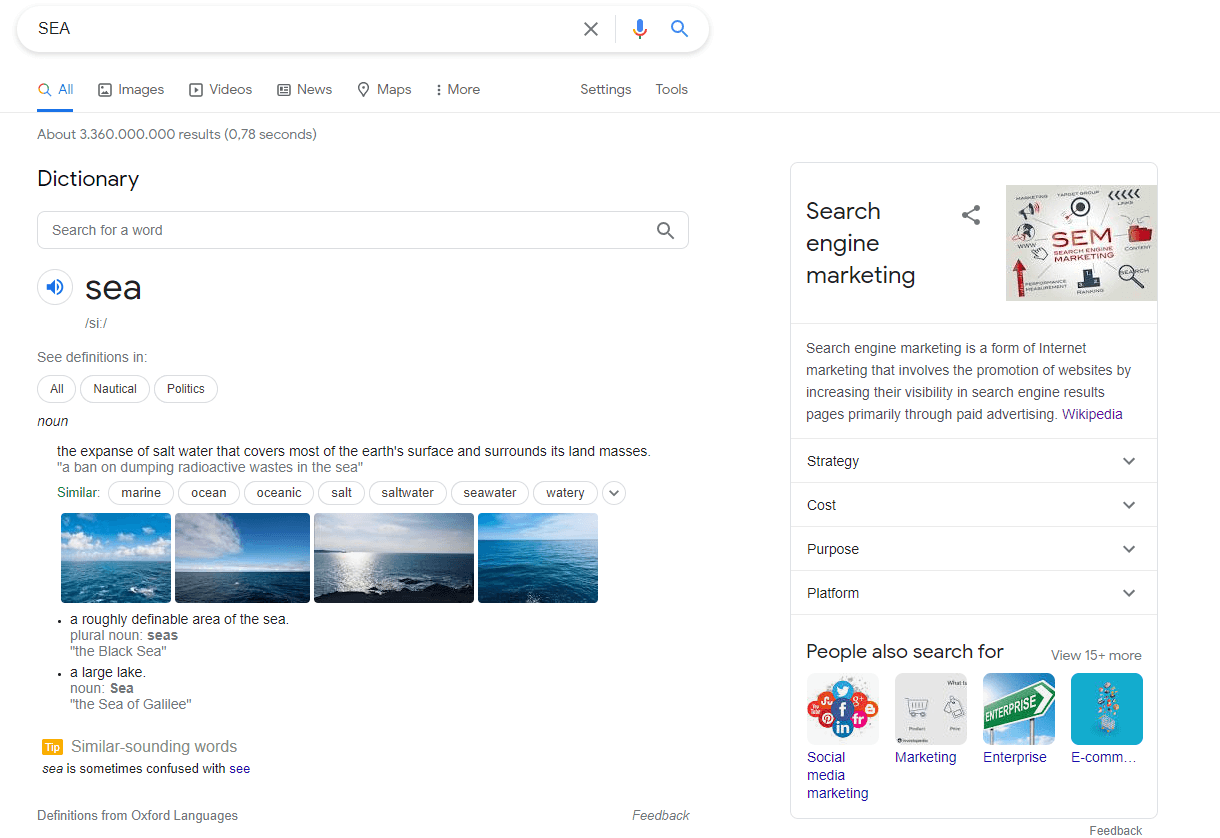At the very top of the image, there is an elongated search box with the text "S-E-A" typed in all capital letters. To the right of this search box, there are three icons: a grey "X" for clearing text, a blue microphone symbol, and a blue magnifying glass symbol indicating a search function. Directly beneath this search bar, the word "All" is underlined in blue, signifying it is selected. Adjacent to "All" are the options: "Images," "Videos," "News," "Maps," and "More." 

Approximately four inches to the right, the words "Settings" and "Tools" are displayed. Below this navigation menu, the word "Dictionary" appears in bold black text. Underneath "Dictionary," there is another search bar with placeholder text "Search for a word," paired with a blue speaker icon to its right. To the right of the speaker icon is the word "C-S-E-A." 

Beneath this search input field, the term "noun" is indicated, followed by a dictionary definition. Supplementing the definition, there are four separate boxes each containing images of the ocean with the sky in the background. 

On the right side of the image, there is a long box titled "Search Engine Marketing," accompanied by selectable links: "Strategy," "Cost," "Purpose," and "Platform." A section titled "People also search for" is listed below these options. At the bottom left corner, there are additional links: "Social Media Marketing," "Marketing," "Enterprise," followed by a prominent blue box labeled "e-com."